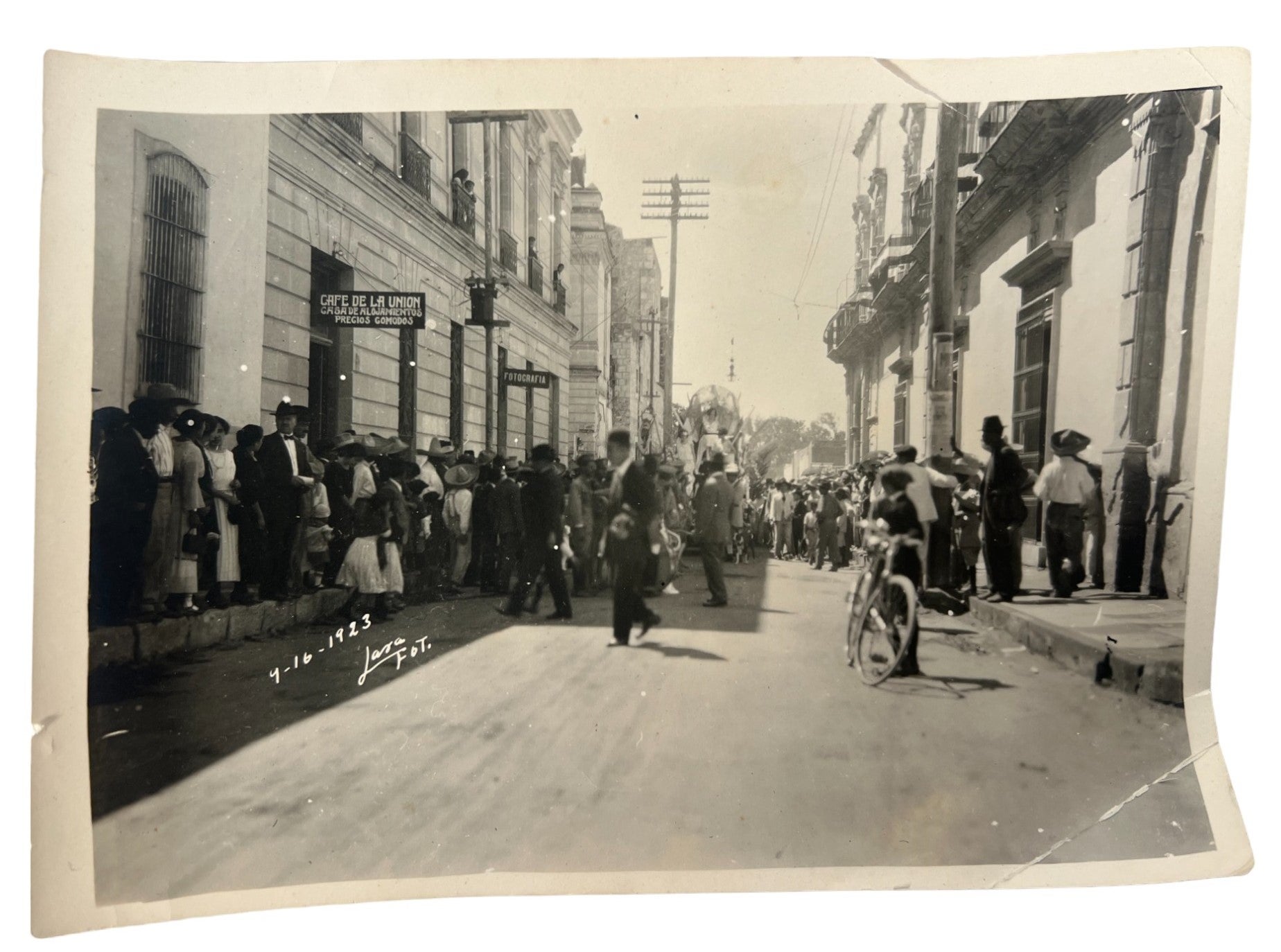This vintage black and white photograph, dated April 16, 1923, portrays a bustling city street scene, potentially in a Spanish-speaking locale, during a parade. The street is lined with well-dressed spectators, men donning suits and hats, while women are also impeccably attired. The crowd, comprising mainly African-American individuals, is densely packed on both sides of the street and on balconies of the surrounding buildings. A sign extending from a building reads "Cafe De La Union," though the rest of the text is partially obscured. In the midst of the activity, a cart with people on it is approaching, and a man can be seen sitting next to his bicycle, looking back at the parade. The photograph, although slightly bent and damaged, captures the anticipation and excitement of the event, frozen in time and framed between telephone poles and characteristic city architecture.